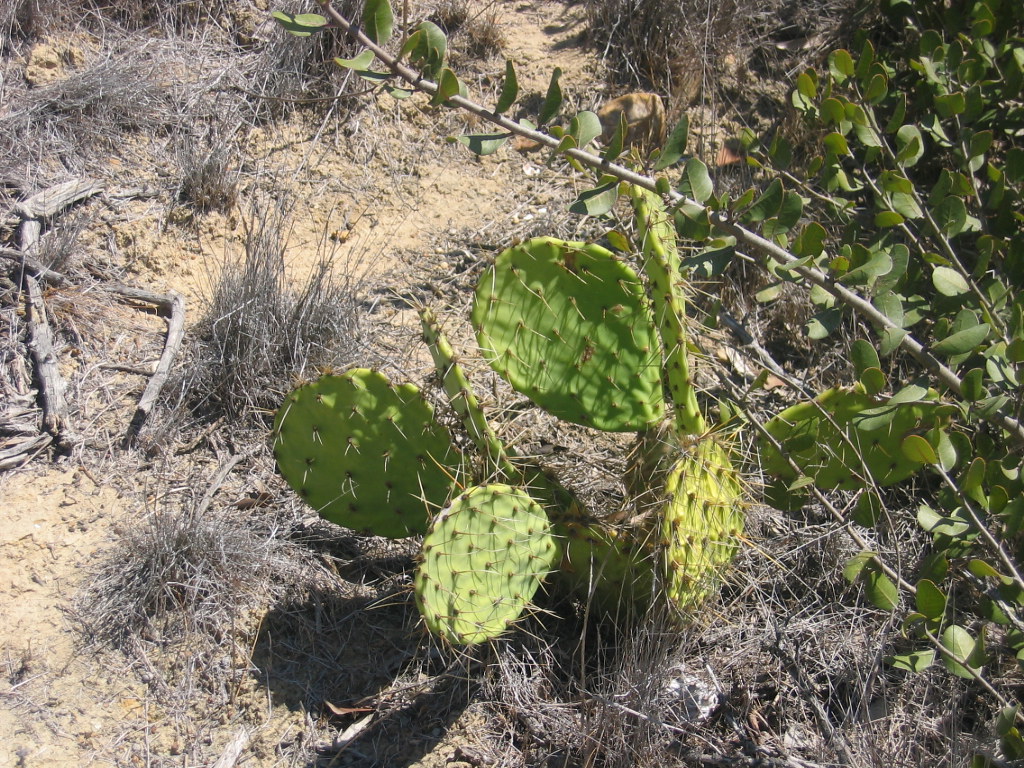In this outdoor photograph, the focal point is a squat, short cactus with seven paddle-shaped, green pads covered in spiky thorns. The cactus stands amidst a barren landscape dominated by sparse, dried grass, brown dirt, and coarse, white to tan shrubs that peek out from the ground. On the left side of the image, some brown sticks and branches are scattered around, and the right side features green leaves on branches, likely part of a tree extending towards the top center of the photo. The scene, bathed in bright sunlight, evokes the arid, dry conditions typical of a desert environment. The overall impression is one of stark, rugged beauty, showcasing the resilience of life in harsh climates.